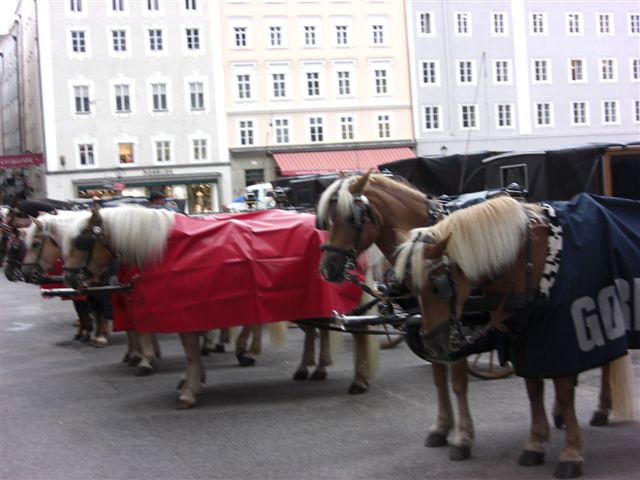In this detailed outdoor photograph, a bustling street corner is prominently displayed, featuring an intriguing blend of architectural and equestrian elements. Central to the image is a white stone building adorned with numerous dark windows, each outlined by a crisp white trim subdivided into six smaller panes. A bright red awning marks a focal point on the building, under which a truck is partially visible, parked on a gray concrete lot.

In the foreground stands a captivating row of light brown horses, each draped in protective coverings. One horse sports a blue sheet adorned with illegible Asian-style text and the partially readable acronym "G-O-B" in white font. Another horse stands out in its striking red sheet. The horses, positioned from the bottom right corner extending to the upper left, include a mix of coats in red and blue, with their milky white manes distinctively flowing.

Accompanying the horses in this vibrant outdoor scene are stagecoaches, enhancing the sense of a historical tableau. The setting is further enriched by the colorful backdrop of an assortment of buildings—apartment homes painted in shades of green, yellow, and purple, adding a whimsical touch to the structured environment. The picture, framed in a square rectangular shape, captures a vivid snapshot of a moment where modernity and rustic charm harmoniously collide.